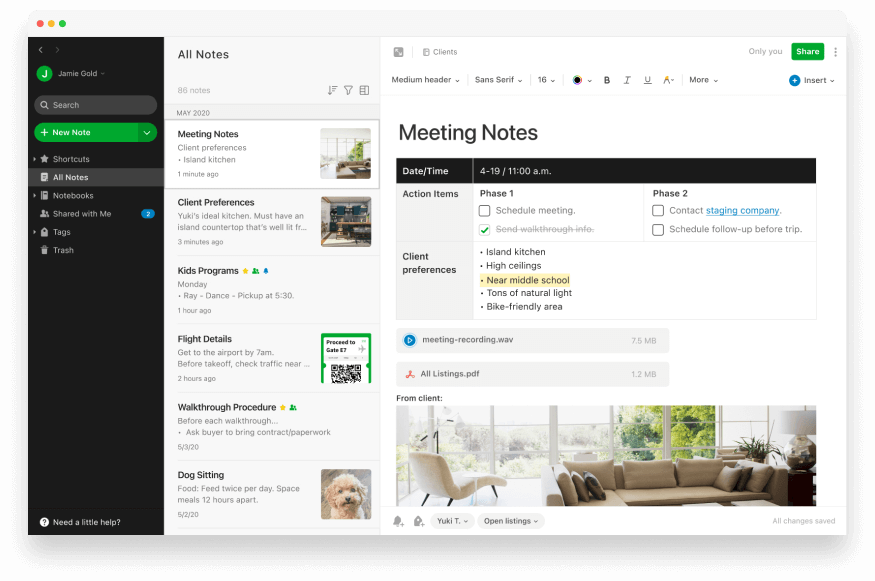The image depicts a webpage from a note-taking application interface. At the top, there is a section with a black background featuring a green circle with the letter "J" and the name "Jamie Gold" beside it. Adjacent to this, there is a search box and a prominent green "New Note" button. The sidebar on the left includes various sections such as Shortcuts, All Notes, Notebooks, Shared with Me, Tags, and Trash.

In the "All Notes" section, there are 86 notes listed, each with different dates. The notes are categorized by month, with the header "May 2020" at the top. Notable entries under this header include "Meeting Notes," "Client Preferences," and "Island Kitchen."

One of the notes titled "Client Preferences" details that Yuki's ideal kitchen must have a well-lit island countertop. Each note is displayed against a white background.

The main section of the page shows a detailed view of a note titled "Meeting Notes," complete with a date, time, and various sections such as action items and client preferences. This note includes an embedded PDF, images from the client, and several tags for easy categorization.

The website or app features a primarily white background with black accents on the sidebar and includes a variety of icons and customization options, indicating a versatile and user-friendly note-taking platform.